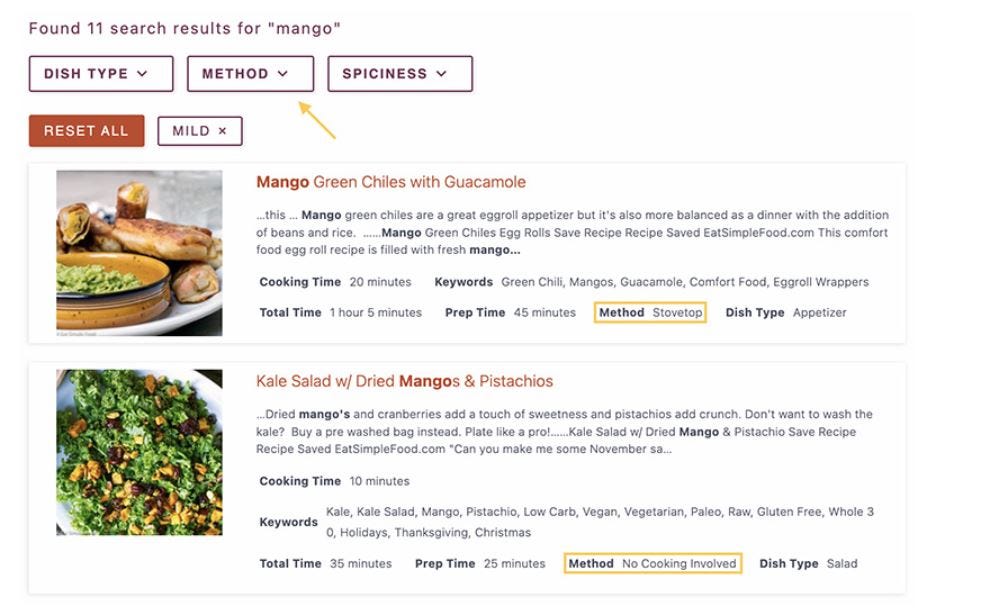The image displays a section of a recipe website. At the top, there are filters for 'Dish Type', 'Methods', and 'Spiciness', with options such as 'Reset' and 'All Mild'. An arrow is pointing at the 'Method' filter. Below, there is a highlighted recipe titled "Mango Green Chilies with Guacamole," accompanied by a vibrant image of the dish. Further down, another recipe is showcased: "Kale Salad with Dried Mangoes and Pistachios," also featuring a picture. Each recipe includes a brief description, about a paragraph long, written in an eye-catching orange font, providing a succinct overview and ingredients.